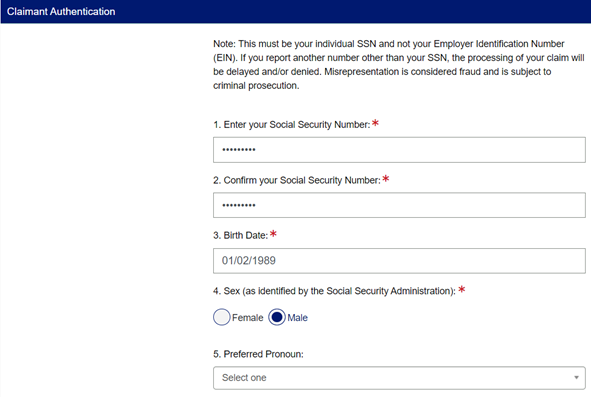A cropped screenshot depicting a section of a claim form focused on claimant authentication. The top of the form features a blue banner that extends horizontally across the page, identifying the section title, "Claimant Authentication." Towards the center-right of the banner, there is an important note highlighting that the individual's Social Security Number (SSN), not their Employer Identification Number (EIN), should be reported to avoid delays or denial of the claim. It also warns that misrepresenting this information is considered fraud and subject to criminal prosecution.

Below this banner, the form sequentially requests specific information:
1. An entry field labeled "Enter your SSN."
2. A confirmation field labeled "Confirm your SSN."
3. A field for the claimant's birth date.
4. An entry titled "Sex as identified by the SSA" with two radio buttons underneath labeled "Female" and "Male," with "Male" being selected.
5. A dropdown menu for "Preferred Pronoun," which currently displays "Select one" indicating that no selection has yet been made.